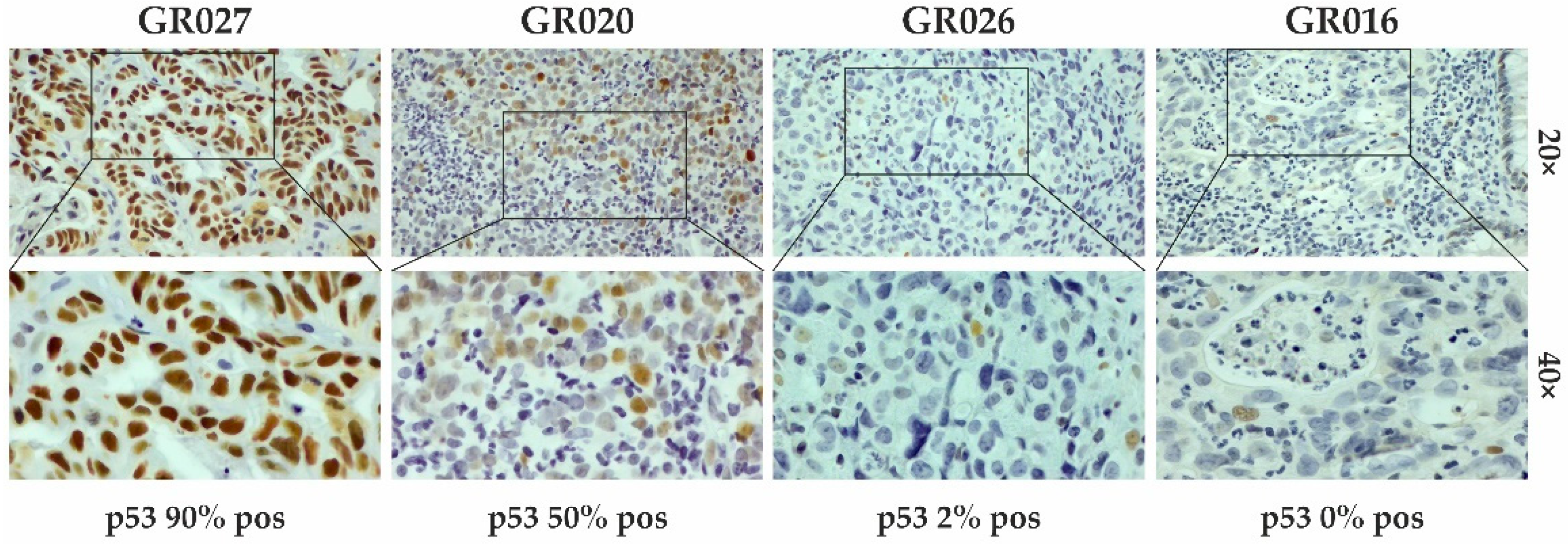The image displays eight rectangular samples, organized in two rows of four, resembling microscopic close-ups of particles. Each sample has corresponding labels at the top and bottom. Above each sample, black text identifiers are present: GR027, GR020, GR026, and GR016 from left to right. Below each sample, the labels indicate measurements of P53 positivity: 90% POS, 50% POS, 2% POS, and 0% POS respectively. The leftmost samples, labeled GR027, display densely packed brown particles, while GR020 contains a mixture of blue and orange particles. GR026 features various shades of blue particles, and GR016 shows primarily blue particles with occasional brown ones. Additionally, the right-hand side of the image notes the magnification levels of 20X for the top row and 40X for the bottom row, illustrating the varying degrees of close-up views. The overall background is white, highlighting the details in these colored particle patterns.